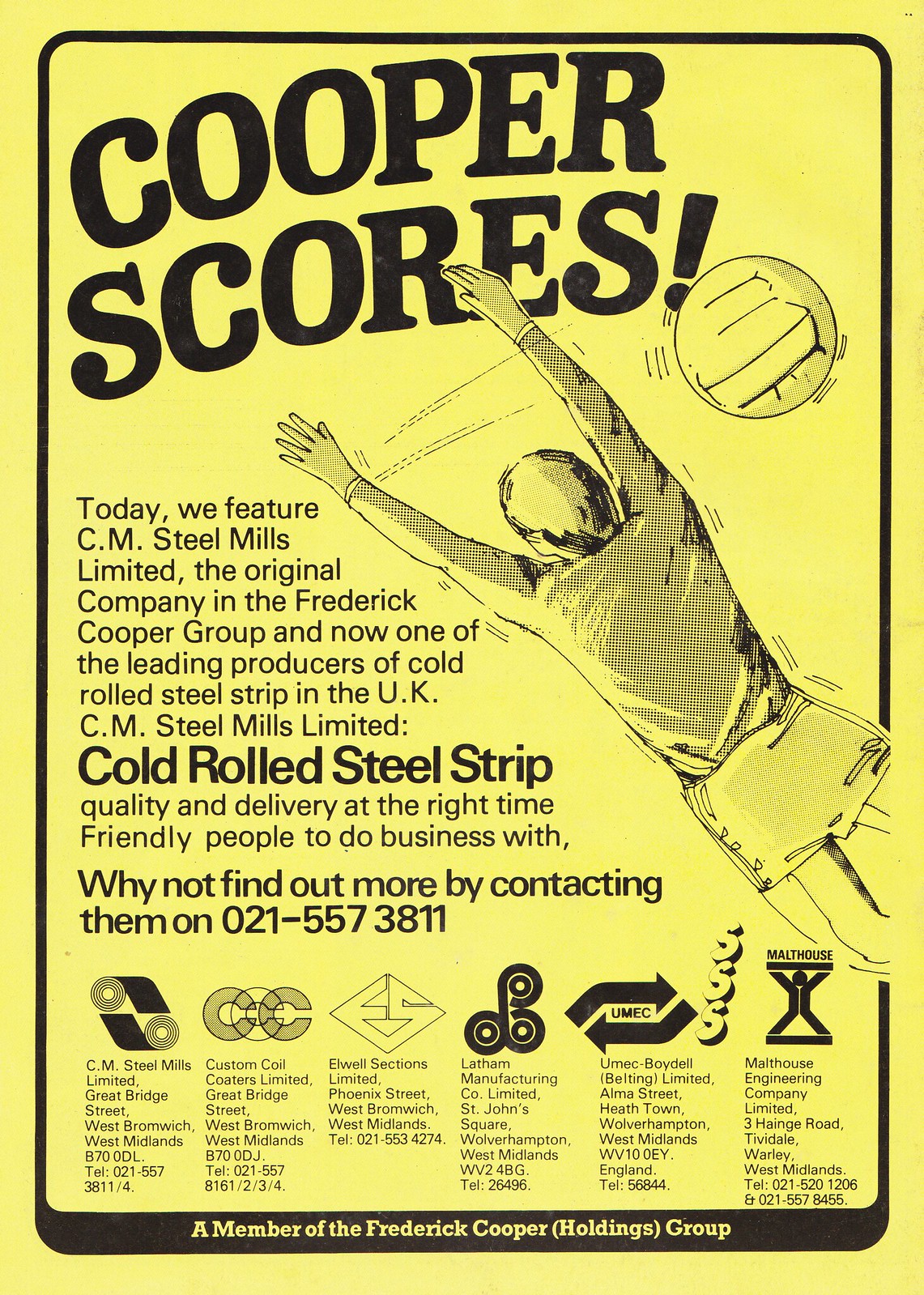The poster, titled "Cooper Scores," has a vibrant yellow background with a black border. Dominating the left side, the poster features detailed text promoting CM Steel Mills Limited, highlighting its prominence as part of the Frederick Cooper Group and its leading role in producing cold-rolled steel strips in the UK. The text emphasizes quality, timely delivery, and friendly service, punctuated by a call to contact them at 021-557-3811.

On the right side, there's a sketch of a soccer player energetically jumping with both hands raised, capturing an action-packed moment. A soccer ball floats nearby, enhancing the sport theme. At the bottom of the poster, a final note proudly states, "A member of the Frederick Cooper Holding Group."